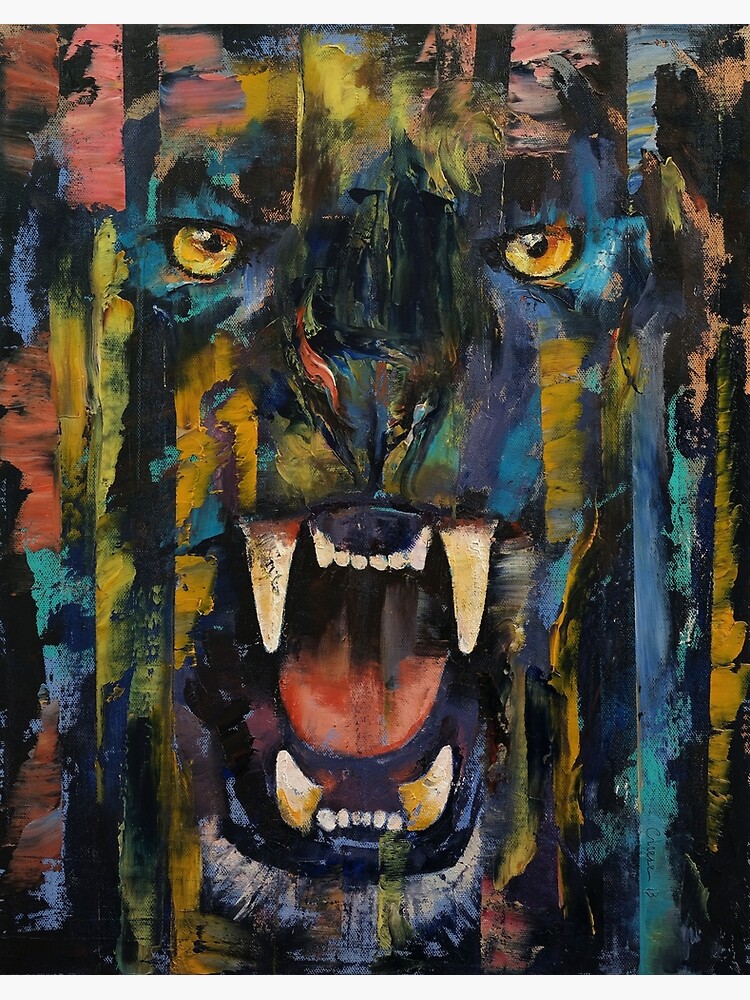This rectangular painting, oriented vertically, depicts a stylized representation of a large cat with its mouth open, showcasing sharp fangs on both its upper and lower jaws. Positioned almost in the center, the cat's nose is clearly visible, while its piercing yellow eyes with black pupils are situated closer to the top of the image. A series of vertical lines in various colors, including yellow, blue, black, red, orange, and brown, dominate the piece, running from left to right and adding a vibrant, abstract quality to the artwork. The combination of these vivid hues and the linear pattern makes it challenging to identify the specific species of the cat.